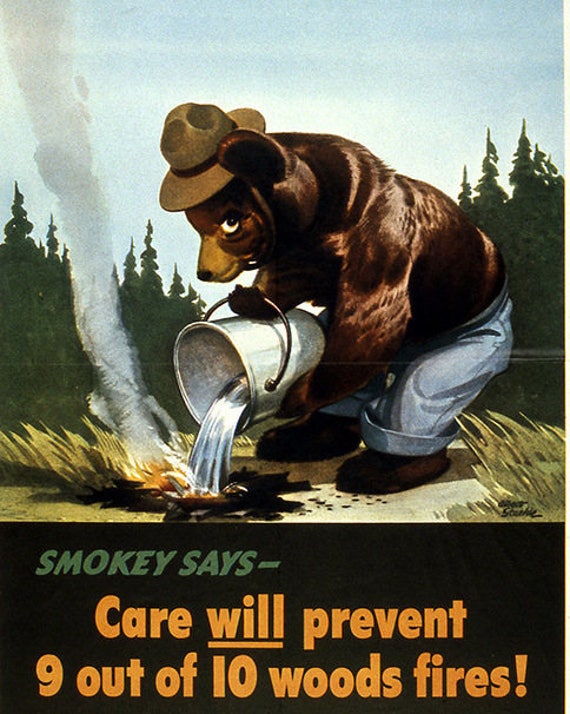The poster, likely from the 1940s or 1950s era, features an older rendition of Smokey Bear. Smokey is depicted without a shirt, clad in blue jeans with rolled cuffs, and wearing his signature tan ranger hat with a black band. He is shown standing amidst a forest background of pine trees and green grass, with a hint of a lake and blue sky in the distance. At the bottom quarter of the image, a black bar contains the text "Smokey says" in green, followed by "Care will prevent nine out of ten woods fires!" in bright orange letters, with an exclamation mark. Smokey is bending over, attentively pouring water from a silver pail onto a campfire that is still smoldering with small flames and smoke billowing up. His gaze is directed towards the viewer, emphasizing his vigilant role in forest fire prevention. The image includes a barely legible signature, possibly reading “Grant S.”, indicating the artist of this classic and diligent reminder to care for our forests.